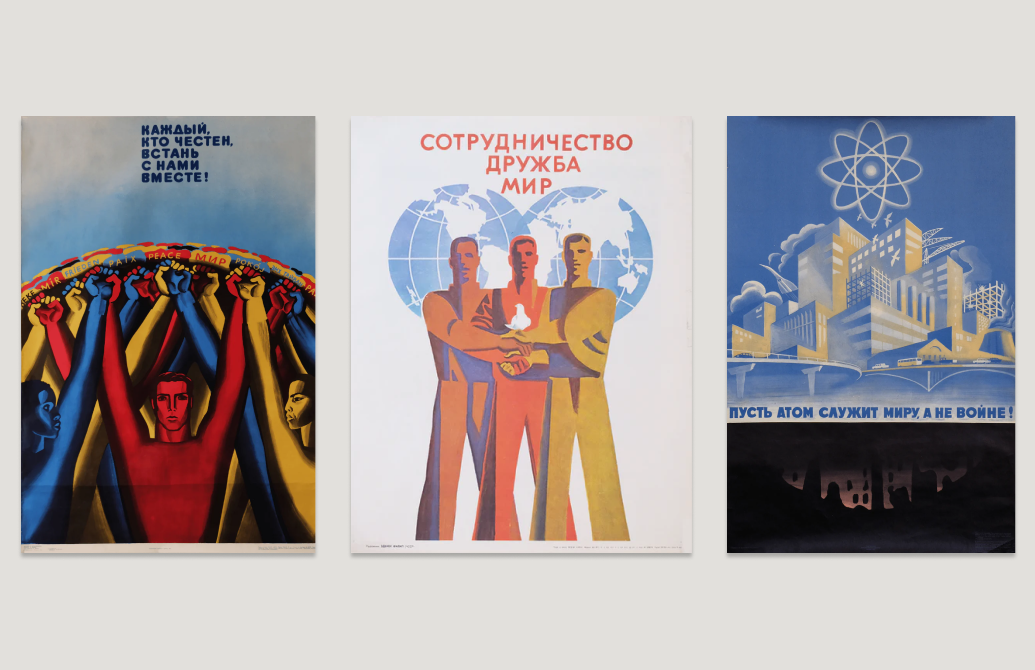The image displays three modern art posters arranged horizontally on a light gray wall. Each poster is a vertical rectangle showcasing unique yet connected themes. The leftmost poster features a blue sky with scattered clouds, showing rows of animated characters from the chest up. These characters, rendered in vibrant hues of red, blue, and yellow, have their hands raised and clasped together under a red, yellow, and blue circular emblem. Unreadable text in a foreign language tops this lively scene. The middle poster portrays three men standing side by side, each in pastel shades of dark orange, red, and yellow, holding hands. They are set against a backdrop featuring two blue globes with white land masses, and a white dove held among them. The rightmost poster depicts a blue cityscape with a centered white moon, crowned by a yellow star, possibly accompanied by an Olympic symbol. Below the city, dark sections interspersed with soft brown geometric shapes dominate, featuring additional unreadable blue text.